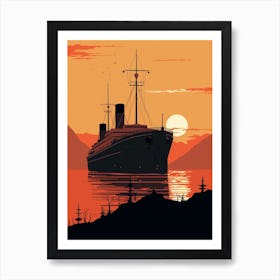A striking piece of art is featured in this image, characterized by a large ship anchored in a bay at sunset. The ship, depicted in dark browns and shadowy tones, exudes an aura of historical grandeur with its two towering masts and prominent smokestacks, yet no sails are visible. The water beneath reflects the warm orange hues of the setting sun, casting a serene glow over the scene. In the foreground, a black, shadowy landscape suggests a shoreline, adding depth to the composition. Distant hills recede into varying shades of red and orange, enhancing the ambiance of a tranquil evening. The setting sun appears as a round, white orb on the horizon, emphasizing the late hour of the day. The overall color palette leans heavily on warm tones, with rich oranges and dark reds dominating the piece. This painting, framed by a black border against a white wall, provides a stark, elegant contrast that accentuates its vivid earthy colors and silhouetted forms. The artistic rendering, devoid of intricate details but rich in atmospheric depth, captures the simplistic yet powerful essence of a bygone era's maritime scene.